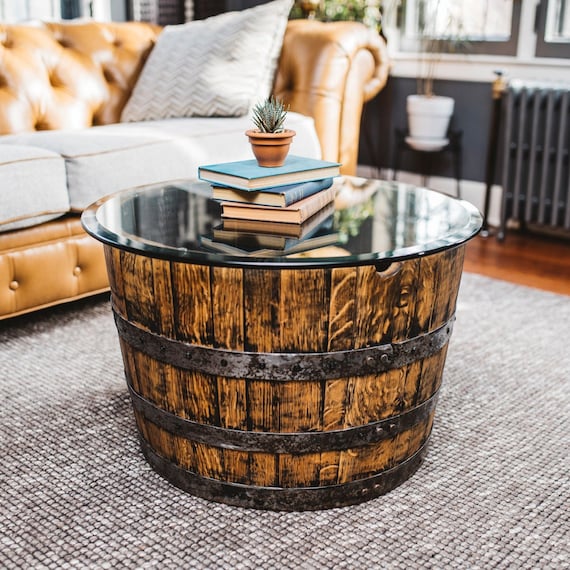This image features a tastefully staged living room with a close-up focus on a distinctive coffee table. In the foreground, atop a textured gray rug, sits a unique table constructed from what appears to be the lower section of a weathered wooden barrel. The barrel is stained in a rich, dark hue and encircled by metal bands, giving it an aesthetically pleasing vintage patina. A round glass piece serves as the tabletop, upon which lie three hardcover books stacked neatly with a small potted cactus on top, adding a touch of greenery.

Background details reveal a sophisticated room painted in gray with white trim, including a set of white-trimmed windows and visible heating vents. A tufted brown leather couch adorned with gray fabric cushions and an assortment of gray patterned pillows stands prominently against one wall. The hardwood floor peeks out from beyond the rug, further highlighting the room's elegant decor. Additionally, blurred in the background, are elements such as ficus trees, a small stand with a white pot, and a radiator, contributing to the room's cozy and lived-in ambiance.